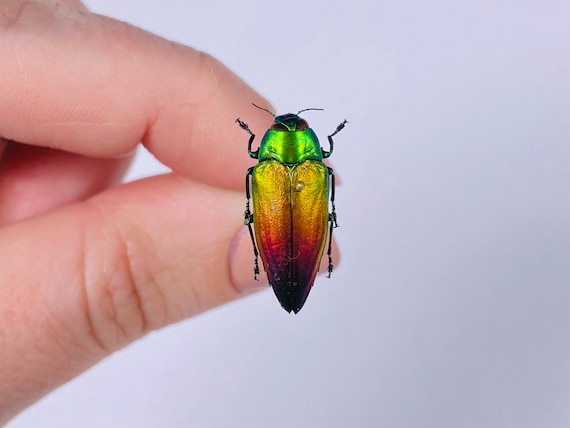In this indoor close-up photograph, a hand emerges from the left side of the frame, with the thumb and index finger delicately holding a small but striking beetle. The background is a pristine white, highlighting the vibrant and iridescent colors of the insect. The beetle's head glows with a neon, shiny green hue, accented by two antennae. Its body transitions from a glittering green-gold around its neck to a golden orange along its wings, which then fade into a rich red, deep purple, and finally, black at the tips. Tiny black eyes are visible on the beetle's head, and it has six legs with two extending near the head, two in the middle, and two towards the back. This captivating beetle with its shimmering, multicolored exoskeleton creates a mesmerizing, almost painted effect as it sits in the fingers of the hand holding it.